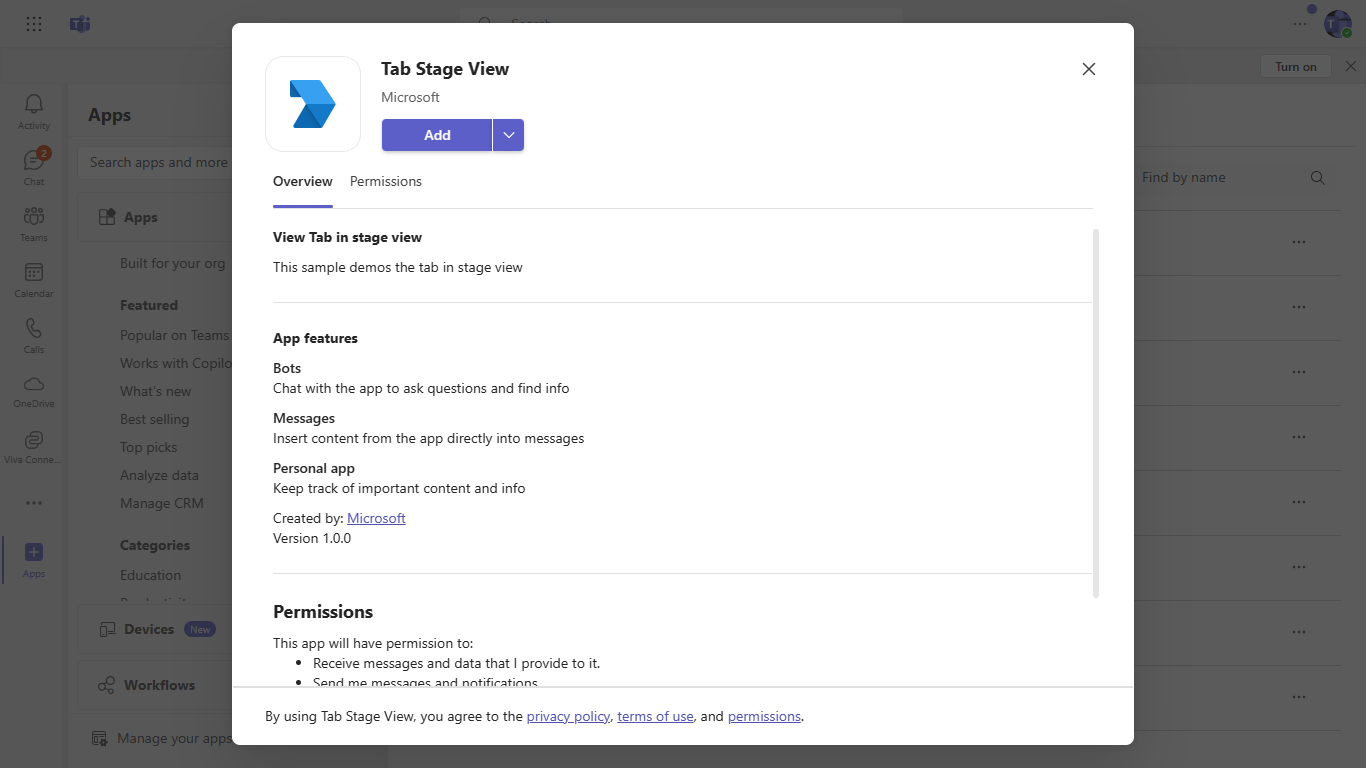The image features a webpage with a gray background overlay, prominently displaying a pop-up box in the center. The popup contains a white square marked with a blue design resembling the tip of an arrow. The heading within the pop-up reads "Tab Stage View, Microsoft" in bold. Below the heading, there's a purple button labeled "Add." Underneath this button, several sections are outlined: "Overview," "Permissions," and a separator line.

Following this, detailed information is provided about the "Tab and Stage View." A brief explanation states, "This simple demo of the Tab and Stage View," with another separator line beneath it. Further down, the "App Features" section lists various functionalities:
- **Box**: Chat with the app to ask questions and find information.
- **Messages**: Insert content from the app directly into messages.
- **Personal App**: Keep track of important content and information.

The app is noted to be created by Microsoft, with the version identified as 1.0.0. 

Another separator line leads to the "Permissions" section, where it specifies that the app has permissions to:
- Receive messages and data provided by the user.
- Send messages and notifications.

It concludes with a statement that by using "Tab Stage View," the user agrees to the privacy policy, terms of use, and permissions.